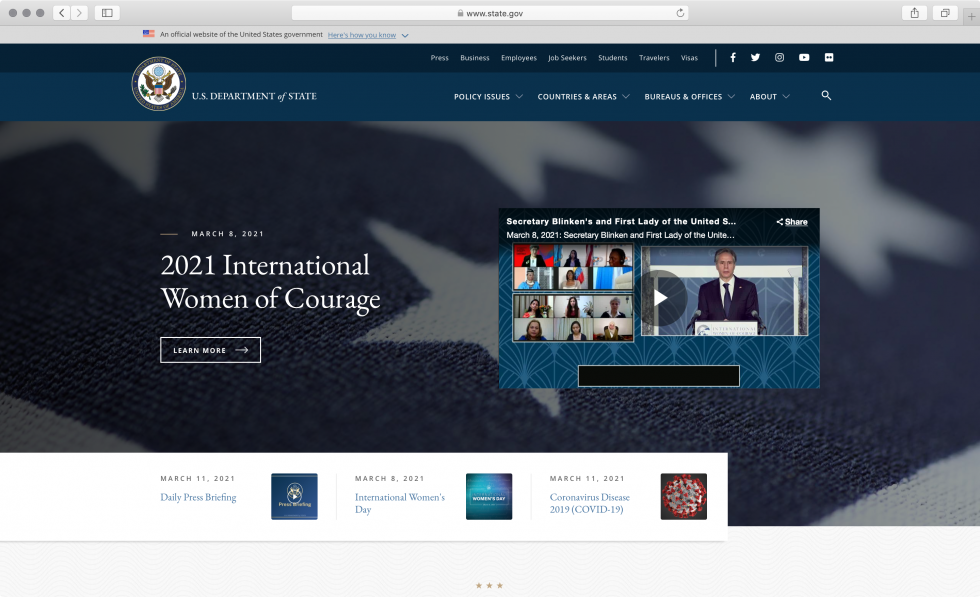This is a detailed screenshot of the U.S. Department of State website as viewed on a Mac computer. The browser's URL bar at the top displays www.state.gov. At the top of the page, there's an official notice featuring an American flag, indicating that this is an official website of the United States government.

Beneath this notice are two horizontal blue bars. The darker blue bar includes navigation links labeled Press, Business, Employees, Job Seekers, Students, Travelers, and Visas. Additionally, there is a vertical separator followed by social media icons for Facebook, Twitter, Instagram, YouTube, and possibly Flickr. On the left side of these bars, overlaying both, is the U.S. government seal, and to its right, the text "U.S. Department of State" is prominently displayed.

The lighter blue bar below includes additional menu items labeled Policy Issues, Countries and Areas, Bureaus and Offices, and About, each accompanied by a drop-down arrow. A search icon, represented by a magnifying glass, is also visible on this bar.

Dominating the page is a large hero image of an American flag in a tight, close-up shot. The focus is on one star in the foreground, with the rest of the stars blurred in the background, emphasizing the intricate details of the flag's stitches. Overlaying the image on the left is the text "2021 International Women of Courage, Learn More." On the right side of the image, there is an overlay featuring Secretary Blinken and the First Lady during what appears to be a Zoom call. Secretary Blinken is seen standing at a podium, and there is an option to play the video.

At the bottom of the screenshot, there is a panel featuring daily press briefings with a video dated March 11th. Other notable entries include coverage of International Women's Day on March 8th and a segment on Coronavirus Disease dated March 11th, accompanied by a 3D representation of the virus.